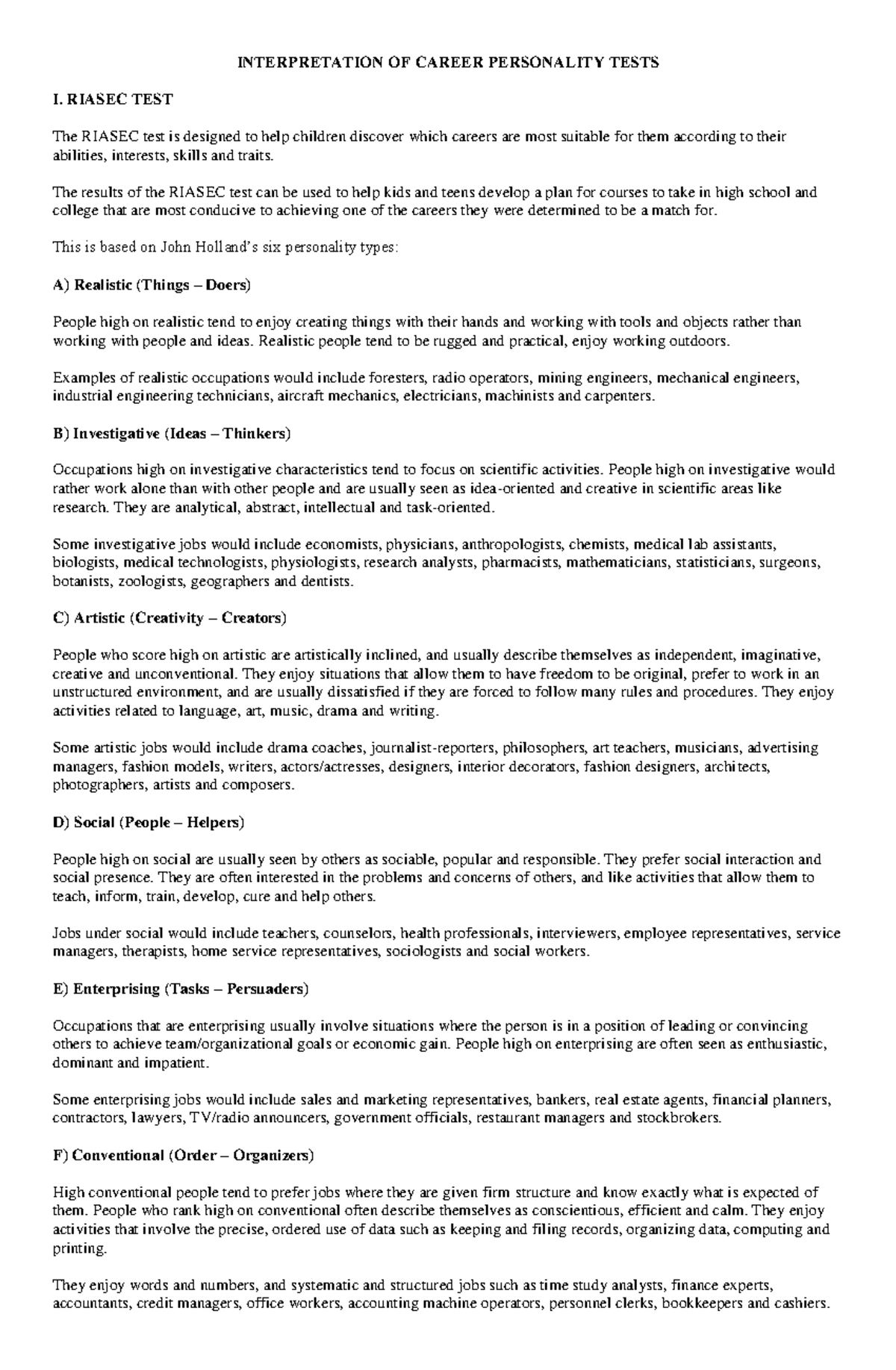### Detailed Caption for Online Article Screen Capture

This image is a screen capture of an online article titled "Interpretation of Career Personalities Test". The article is presented in an outline format, centered around the R-I-A-S-E-C test, which is the first main point of the outline. The R-I-A-S-E-C test is structured based on John Holland's six personality types, and the outline includes several subsections labeled from A to F. 

Each subsection corresponds to one of the personality types:
- **A. Realistic (Doers)**: 
- **B. Investigative (Thinkers)**: 
- **C. Artistic (Creators)**: 
- **D. Social (Helpers)**: 
- **E. Enterprising (Persuaders)**: 
- **F. Conventional (Organizers)**: 

Under each subheading, there are brief descriptions, typically two to three sentences long, explaining the characteristics of each personality type. 

Due to the extensive content, only the structure of the outline is noted here, showcasing an organized framework for understanding different career personalities as interpreted by the R-I-A-S-E-C test.